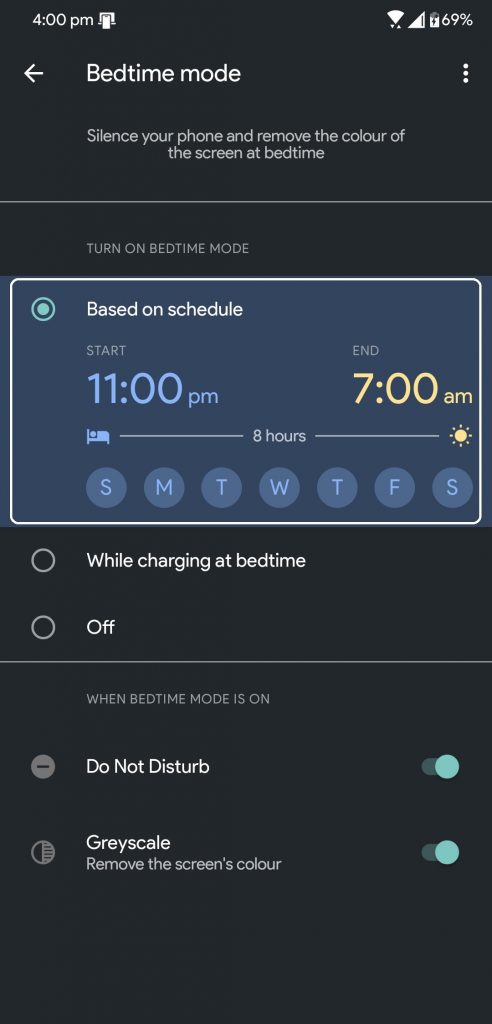The image depicts a cell phone screen displaying a detailed interface related to a Bedtime Mode. Here is a comprehensive description:

At the top left corner, the screen indicates the time as 4 p.m. On the right side, there are icons representing Wi-Fi and cellular signal strength, accompanied by a battery icon showing 68% charge. 

Just below the status bar, a back arrow is visible on the left with the label "Bedtime mode" next to it. On the right, there are three vertically aligned dots, suggesting a menu or additional settings. 

Beneath this header, a brief description states: "Silence your phone and remove the color of the screen at bedtime." 

A horizontal line separates this section from a prompt that reads "Turn on Bedtime mode," followed by a blue-gray rectangular button with white text. This button indicates that Bedtime Mode is scheduled to start at 11 p.m. and end at 7 a.m.

Below the button, there is an icon of a bed with a horizontal line beneath it. In the middle of this line, the text "8 hours" appears, with a sun icon at the line's end, signifying the duration of the scheduled sleep interval.

Following this, there are seven circles representing the days of the week (S, M, T, W, T, F, S). These circles and their letters are a lighter blue compared to the background. The text "Start" is also in light blue, indicating the time at the beginning of Bedtime Mode, and "7 a.m. End" is highlighted in yellow, specifying the wake-up time.

Further down, there is an option titled "While charging at bedtime," with an adjacent circle that is unticked. Below it, there's an "Off" option, which is also unticked. 

A gray dividing line follows, leading into additional settings specifying the effects of Bedtime Mode when activated. It notes that "Do Not Disturb" is enabled, shown by a green-colored indicator with a small circle containing a line through it. Additionally, "Grayscale" mode is toggled on, as indicated by the corresponding setting.

This detailed interface provides users with comprehensive controls for managing their device’s Bedtime Mode, ensuring a distraction-free and restful night’s sleep.